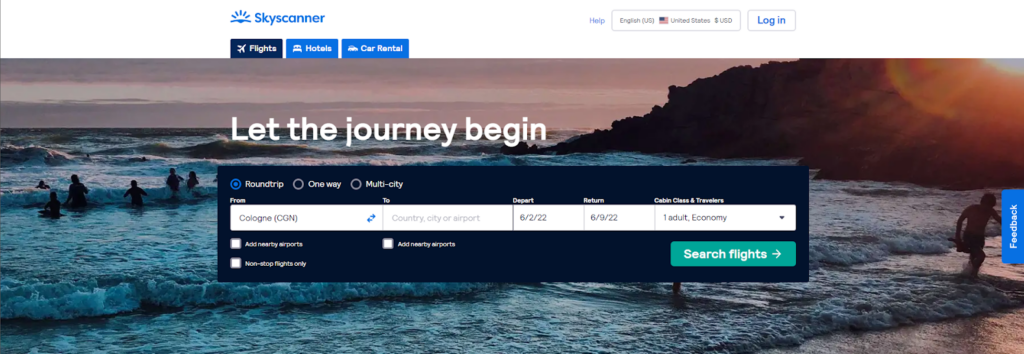This horizontal image, presented by Skyscanner, showcases their branding with a blue sun symbol emitting sun rays. At the top of the image, prominently displayed are the options for "Flights" in black, and "Hotels" and "Car Rental" in blue boxes. A search bar and login option are also visible.

The background features a stunning beach scene during sunset. The sky is gradually darkening, accentuating a gorgeous mountain on the right side. The beach is lively, with people enjoying the water, including a man emerging from the waves.

In the foreground, a pop-up box offers various travel options: "Round Trip," "One Way," and "Multi-City," all in white text. Below this, a white information bar lists the fields for country names, destinations, airports, travel dates, and specifies "one adult, economy." At the bottom of the pop-up, a green "Search Flights" button invites action.

On the left side, smaller white text provides additional information, while the right side features a blue feedback bar for user comments.